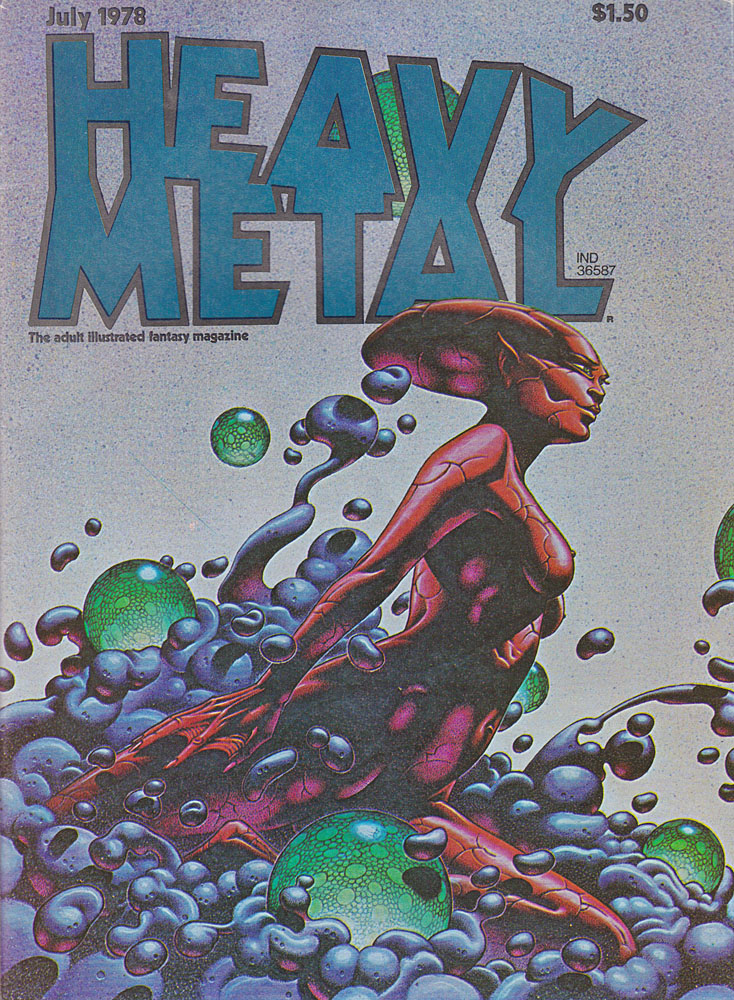The cover of the July 1978 issue of Heavy Metal magazine, priced at $1.50, features a richly detailed, colorful illustration that vividly encapsulates the sci-fi and fantasy themes of the period. The title "Heavy Metal" appears in large, block letters shaded in dark blue and highlighted with black, with the word "Heavy" stacked on top of "Metal" and merging into it. Below the title, in small black type, reads "The Adult Illustrated Fantasy Magazine." The textured background resembles a brick wall, adding depth to the cover.

Dominating the scene is a futuristic, red and burgundy-colored alien woman with webbed hands and intricate lined details, giving her an otherworldly appearance. She seems to be emerging from or interacting with a dark blue, churning liquid filled with inky, soapy bubbles. Floating around her are several green, scaly orbs with small dotted patterns, emphasizing the surreal and fantastical elements of the cover. The illustration captures the vibrant and eclectic spirit of the 1970s, marking it as a standout piece of graphic art from the era.